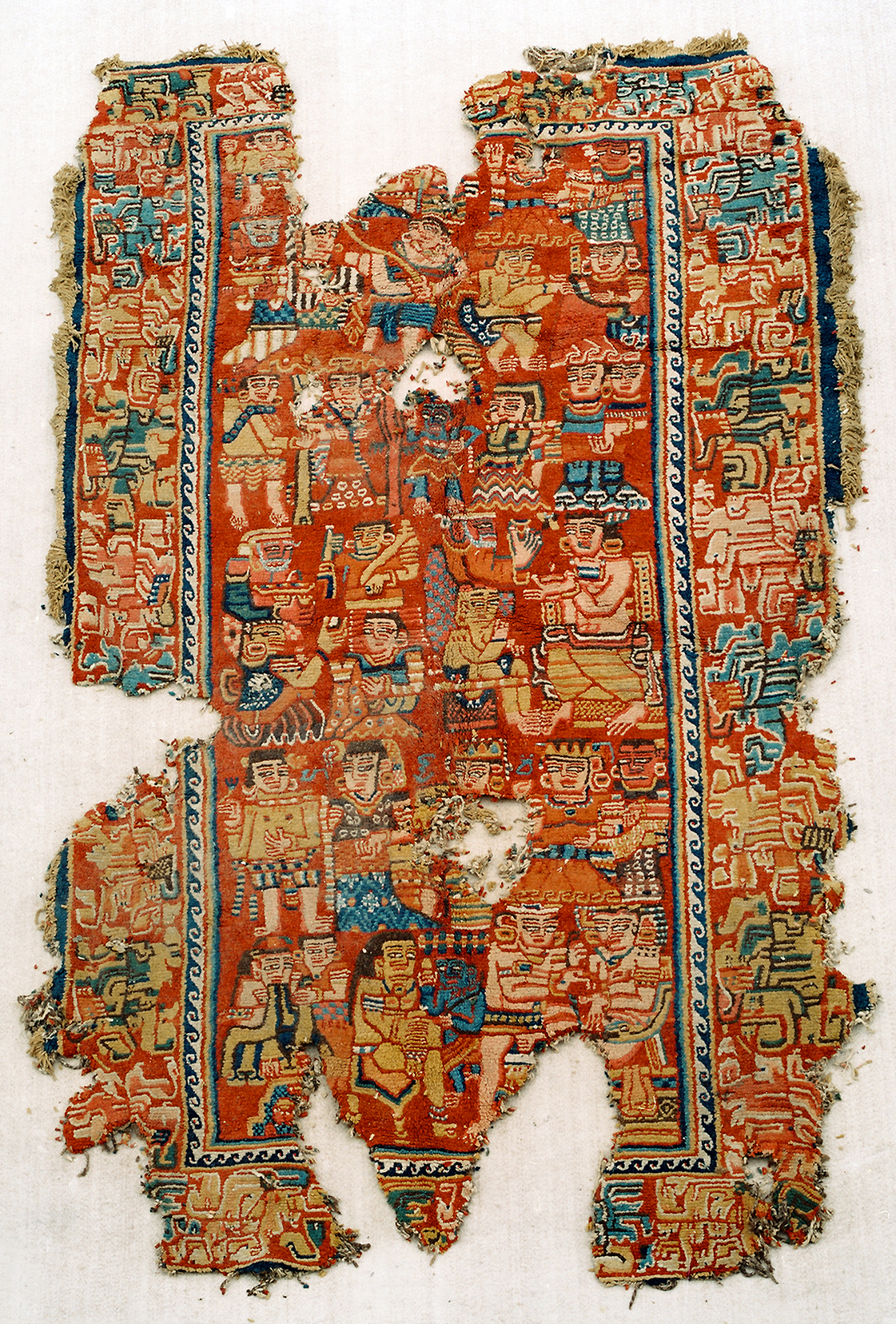This image depicts an old, worn, and tattered tapestry or textile, viewed from the top. The tapestry features a frayed golden fringe that is mostly intact in the top left, top right (though missing an angled corner), and bottom left, but is otherwise torn away in chunks around the edges. The background is predominantly a faded red, with the centerpiece showcasing rows of human characters, roughly five per row, adorned in various traditional garments. Encircling these figures is a rectangular border with a blue and white wave design framed by a yellow stripe, followed by another stripe in red, yellow, light blue, and dark blue. Beyond this central portion, abstract human figures are depicted on a white backdrop. The tapestry has significant damage, with large rips and holes, including a substantial tear almost at the center top, a big rip on the left side middle, and a shoe-sized hole at the bottom. The right side is notably distressed, with a large section ripped away. Despite its disrepair, the detailed artistry suggests influences possibly from Mayan or Aztec cultures, featuring mostly red hues with accents of brown, green, and blue, all faded with age.